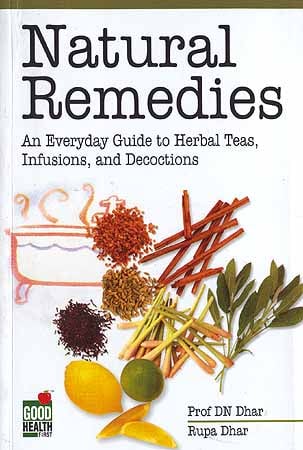The image depicts the front cover of the book titled "Natural Remedies: An Everyday Guide to Herbal Teas, Infusions, and Decoctions" by Professor D.N. Dhar and Rupa Dhar. The book is published by the Good Health Company, as indicated by the logo in the bottom left corner. The cover, which has a white background with black text, features a bathtub with a small amount of water and an assortment of spices and herbs that can be used in baths or infusions. These include turmeric, mint, lemon, lime, pepper, cinnamon sticks, red and brown powders, and various leaves and stems, possibly sage. In addition, there is an image of a cooking pot with steam rising, suggesting the preparation of herbal remedies. The detailed illustrations emphasize the natural ingredients used for these remedies, aligning with the book's content on everyday herbal treatments.